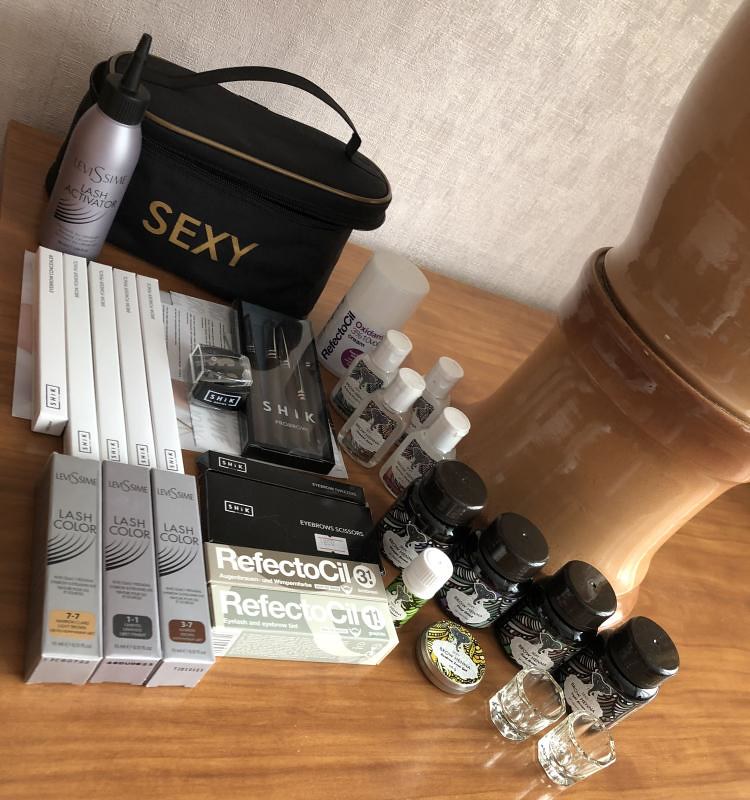In this photograph taken from an angle looking downward, the highly glossy and reflective wooden surface dominates the scene. Off to the right, a planter or vase is prominently displayed, and its clear reflection is captured beautifully in the wood. In front of the vase, there are numerous small bottles and several long, narrow cardboard boxes. 

In the background, an oval-shaped container made of possibly leather and adorned with the word "SEXY" in gold lettering contributes to the array of objects. Adjacent to this container is a lavender-colored bottle labeled "Lash Activator." 

A cluster of white cardboard boxes with unreadable text finds its place next to gray boxes labeled with different lash colors, identifiable by the small colored squares on them. Also in the mix are a few more white cardboard boxes labeled "Reflectocil 3 and 1." 

Above this assortment, black boxes labeled "Scissors" are visible, accompanied by another black box inscribed with "SHIK," containing brushes. Additionally, to the right, there are several small bottles, some with white tops and others with black tops, adding to the detailed and varied collection on display.